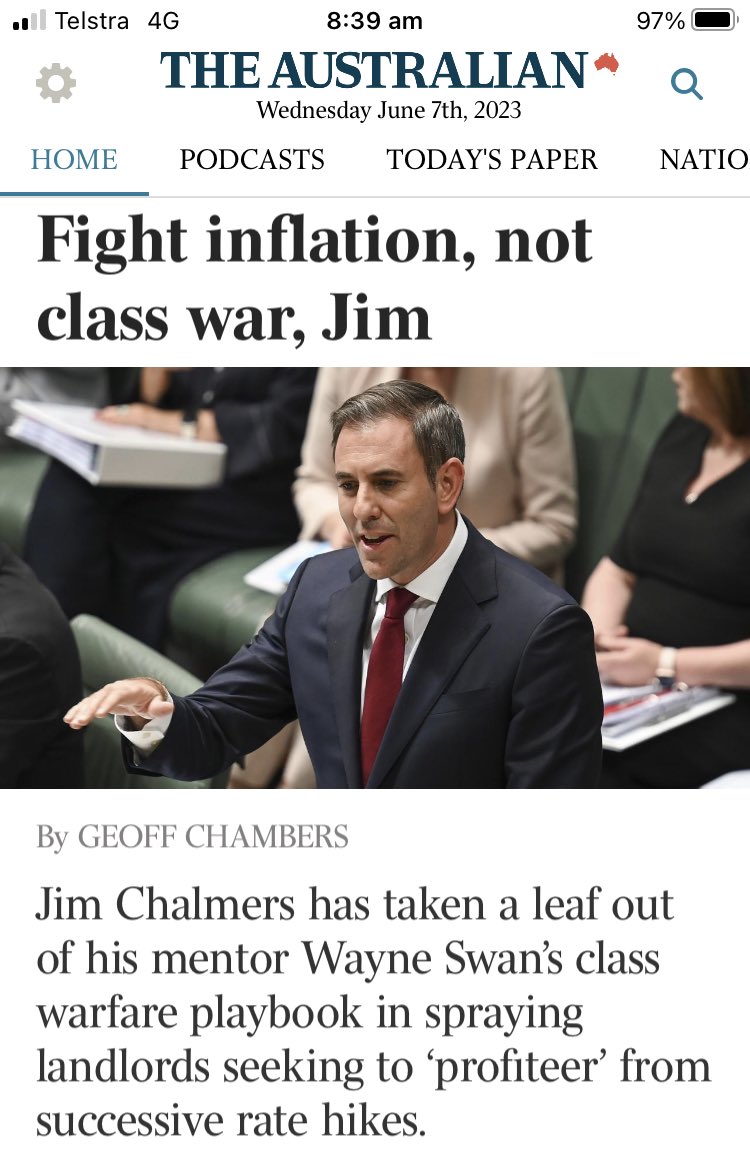A detailed descriptive caption for the given screenshot could be:

---

A screenshot taken from a smartphone display showcasing the current Telstra coverage at 4G with 2 bars signal strength, the time at 8:39 a.m., and 97% battery life. The captured content appears to be from "The Australian," identifiable by its blue-colored title with a red map of Australia logo beside it. The all-caps subheading reads "THE AUSTRALIAN," and the date is marked as Wednesday, June 7th, 2023. 

In the interface, there are options to access settings on the left and a search bar on the right. Main navigation tabs across the top include "Choice," "Home," "Podcast," "Today's Paper," and a partial word "Nashio," with the current selection being "Home."

The headline under "Home" reads "Flight Inflation not Class War" by Jim, accompanied by an image of a politician, dressed formally in a suit, delivering a speech. The article is penned by Jeff Chambers, discussing how Jim Chalmers has adopted strategies from his mentor Wayne Swan's class warfare approach, criticizing landlords for capitalizing on successive rate hikes. The typical rhetoric of politicians dictating financial decisions is highlighted.

---